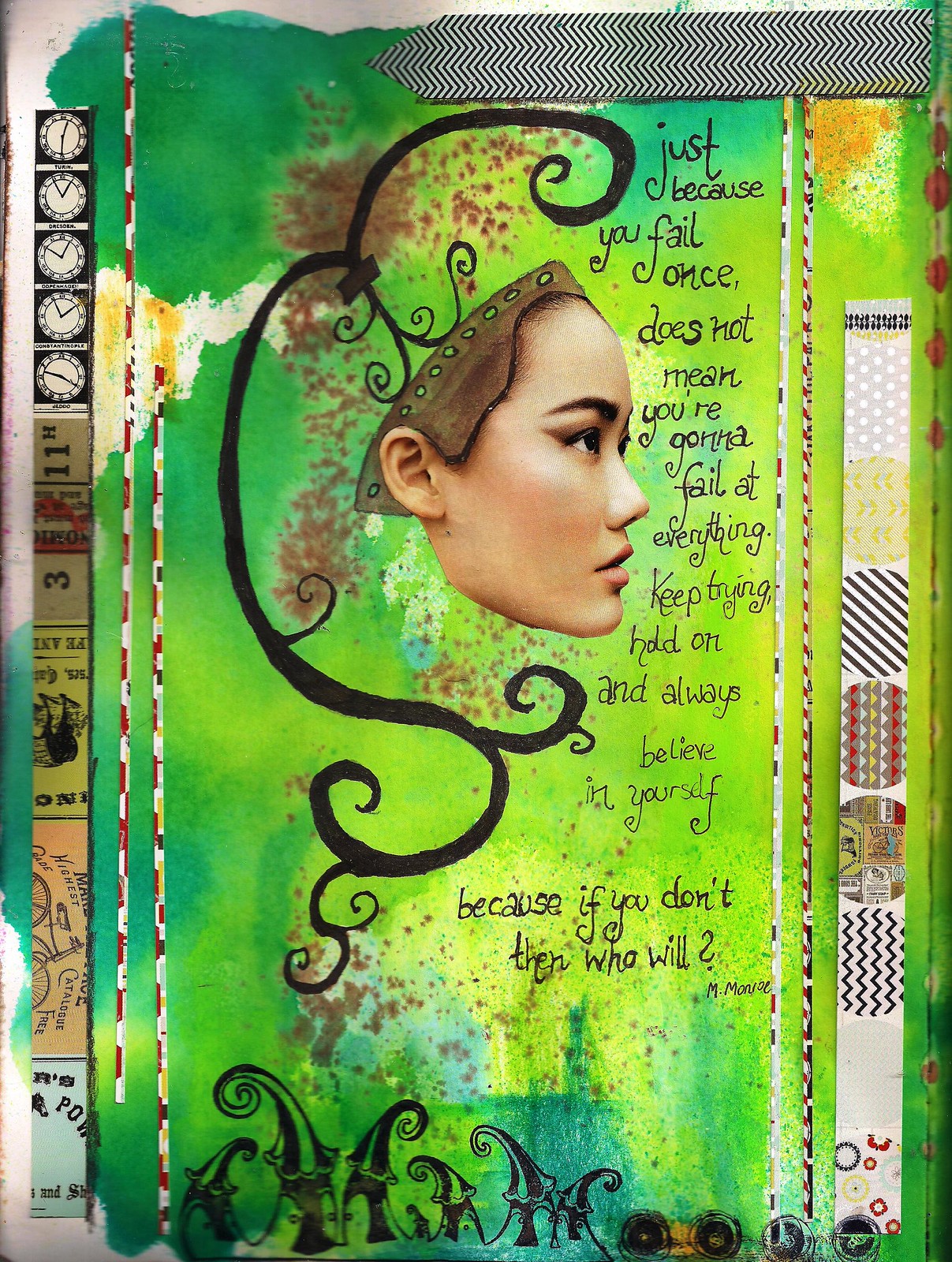This intriguing piece of mixed media artwork features a predominantly green, blue, and yellow color palette with the background appearing as a spotty brown and green watercolor wash. A thin band on the left side presents newspaper advertisement clippings and clocks set within squares. The right side is adorned with a variety of mixed patterns.

At the heart of the composition is the profile of an Asian woman's face, delineated with intricate, curly black vine-like decorations encircling her head, contributing to the ethereal quality of the piece. She appears to wear a brown hairband dotted with little green spots.

Accompanying her profile, handwritten in an elegant script to the right of her face, is an inspirational quote: "Just because you fail once does not mean you're going to fail at everything. Keep trying, hold on, and always believe in yourself, because if you don't, then who will?" This motivational message is attributed to M. Monroe, presumably the iconic Marilyn Monroe. At the bottom, whimsical illustrations resembling little curly circus tents add a playful element to the piece, enriching its overall complexity and charm.